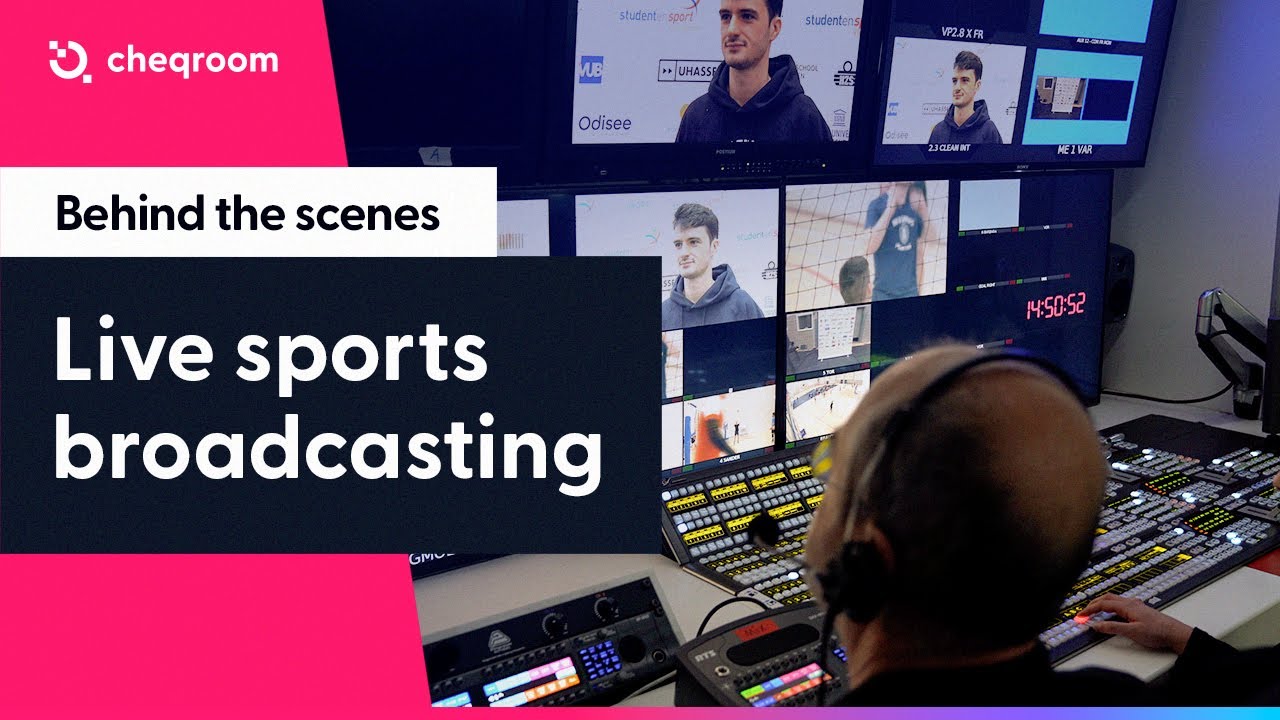This visually striking advertisement for Cheqroom (spelled C-H-E-Q-R-O-O-M) features their distinctive logo in the top left corner, comprising a backward ‘C’ encircled by three dots—two within the ‘C’ and one on its outer edge. The logo is placed against a red or light pink slanted divider. Just beneath the logo, a white banner with black text reads “Behind the Scenes,” followed by a black banner with white text proclaiming “Live Sports Broadcasting.”

On the right side of the image, a balding sportscaster equipped with glasses and a headset with a microphone is intently monitoring an array of screens, showing various camera angles of a live sports event, likely volleyball, indicated by a visible net. In front of him, a sophisticated control panel brimming with numerous dials and switches signifies the technical complexity of managing the broadcast. Additionally, a clock on the dashboard displays the time as 14:50:52:250. Another person's arm rests on a keyboard adjacent to the sportscaster's console, suggesting a collaborative effort in the broadcast control room. The overall composition underscores the intricate and dynamic nature of live sports broadcasting, reinforcing the brand’s expertise in providing behind-the-scenes insights.